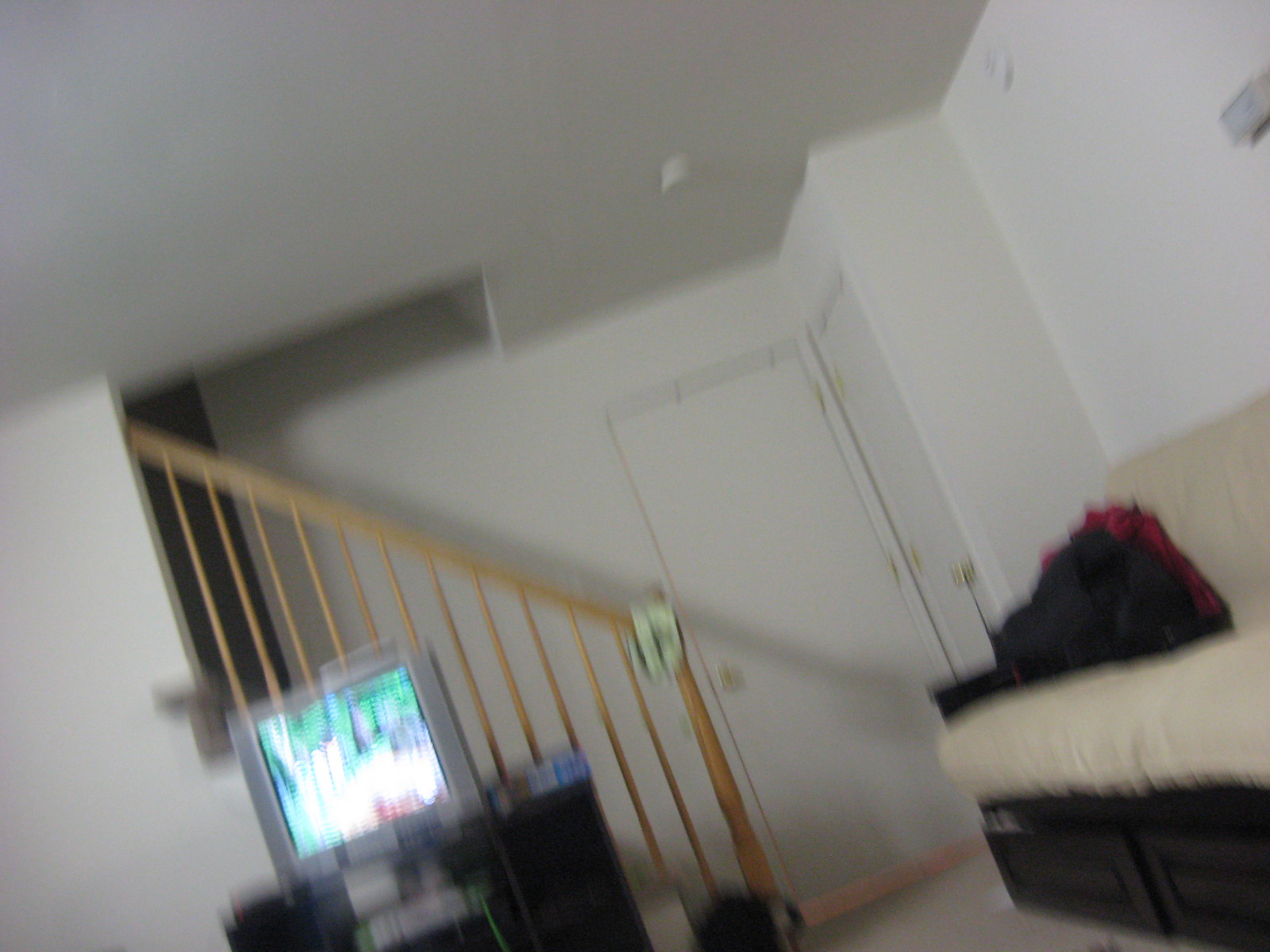The photo captures a well-lit indoor scene, albeit slightly blurry, taken from an angled perspective. Central to the image is a computer monitor, illuminated but displaying indistinct green and white patterns on its screen, suggesting it is powered on but not displaying specific content. The monitor rests on a desk, reinforcing the workspace atmosphere.  

To the right, a wooden bench with a brown padded cushion is visible. A striking red piece of cloth, possibly a garment or small blanket, is casually draped over the bench, adding a splash of color to the otherwise muted scene. 

The room's walls are painted in an off-white hue, contributing to the bright and airy feel. Two closed doors are part of the backdrop, hinting at adjoining rooms or storage spaces. 

On the left side of the image, a wooden banister leads upward, indicative of a staircase. The stairs ascend to a shadowy, partially obscured hallway at the top, adding depth and a sense of intrigue to the composition. Overall, the room appears to be a blend of functional workspace and casual seating, captured in a slightly blurred yet descriptively rich photograph.